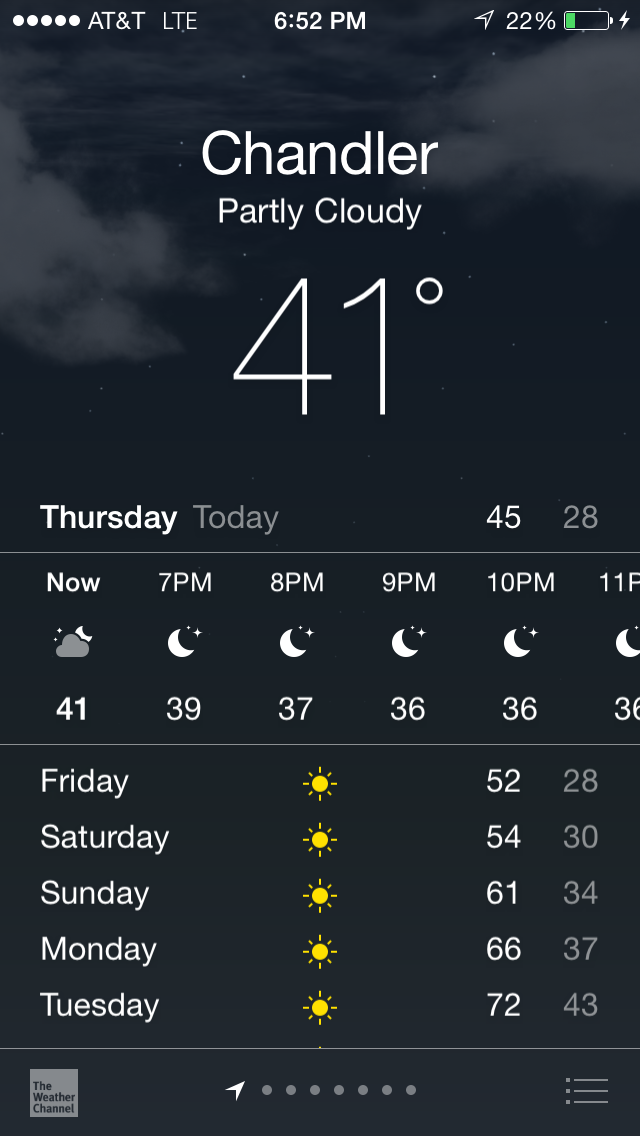This is a detailed caption of an image depicting a weather forecast screenshot on a smartphone, set against a nighttime sky backdrop. 

The sky is a dark bluish hue with hints of blue and white clouds in the top left and right corners. At the very top, five white dots are visible, followed by "AT&T LTE," indicating the network status. Centrally, it reads "6:52 PM." To the far right, there's a white upward-pointing arrow indicating a 22% battery charge, accompanied by a battery icon and a lightning bolt, suggesting it's charging.

In the center of the screen, the text "Invite Chandler" is displayed, followed by "Partly Cloudy" and a temperature of "41°," with a degree symbol. Below that, "Thursday" is noted, labeled as "Today" on the right. Adjacent to this, the temperatures 45° and 28° are stated, indicating the high and low for the day.

A timeline runs horizontally across the screen, displaying the time slots: Now, 7 PM, 8 PM, 9 PM, 10 PM, and 11 PM. Each time slot is depicted with consecutive images of five crescent moons. Below these icons are corresponding temperatures: 41°, 39°, 37°, 36°, and 36°. 

A gray line separates this section from the daily forecasts listed vertically: 
- Friday: 52°/28° 
- Saturday: 54°/30° 
- Sunday: 61°/34°
- Monday: 66°/37°
- Tuesday: 72°/43°

Icons of a yellow sun accompany each day's forecast.

In the bottom right corner, there's a white box labeled "The Weather Channel" in black text. Adjacent to this box are seven gray dots and an upward-pointing white arrow. Below these are three vertically-arranged dots, each with a horizontal dash.